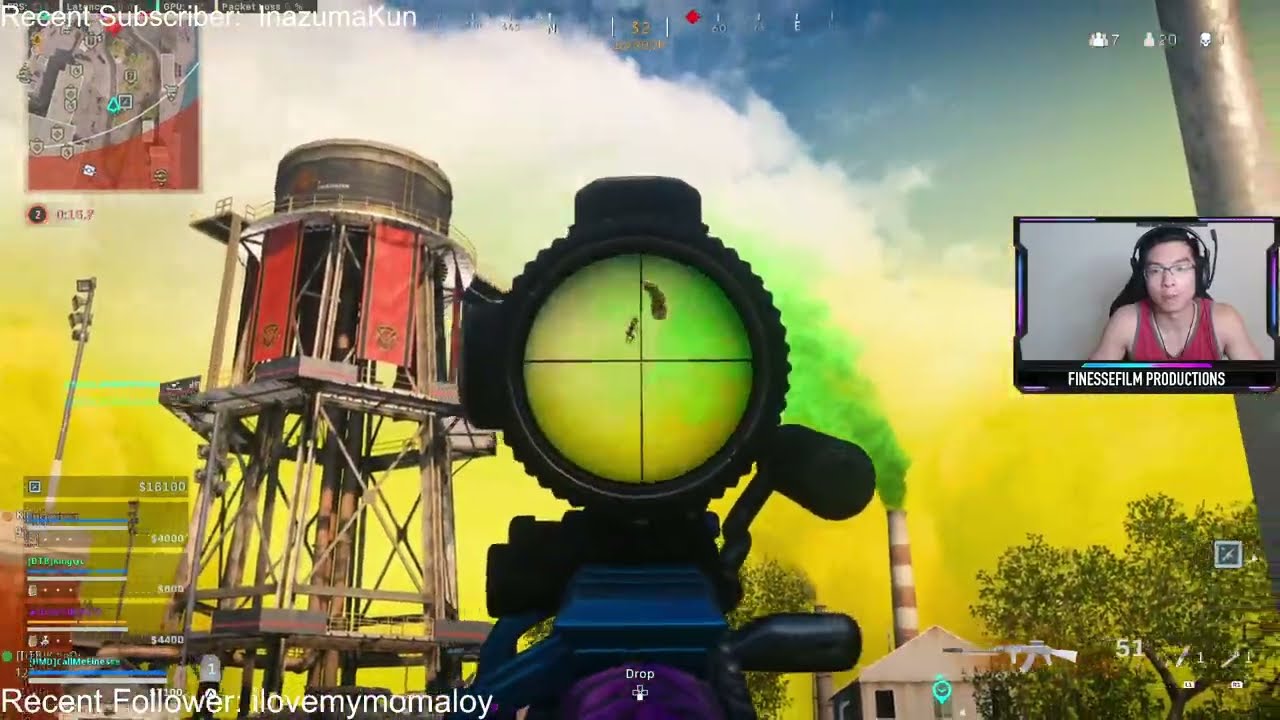The image is a detailed screenshot from a first-person shooter video game, capturing an active gameplay moment. At the center of the screen, you can see the player's gun with crosshairs targeting a descending parachuter. To the right of the gun is the player's webcam feed, showing a man wearing over-the-ear headphones and glasses, possibly a streamer, dressed in a red tank top. Beside this, in white text, it reads "Finds Film Productions."

The top left-hand corner features a mini-map of the game, below which score details are visible, along with a compass at the top. The environment in the background displays a large water tower and a plant emitting green smoke, set against yellow mustard clouds, accompanied by a few trees. The bottom left of the screen shows colored bars, possibly indicating follower activity with the text "recent follower I love my mama Loy," highlighting the active stream. In the bottom right-hand corner, there's information about the gun and its ammunition, cementing it as a live gameplay snapshot.